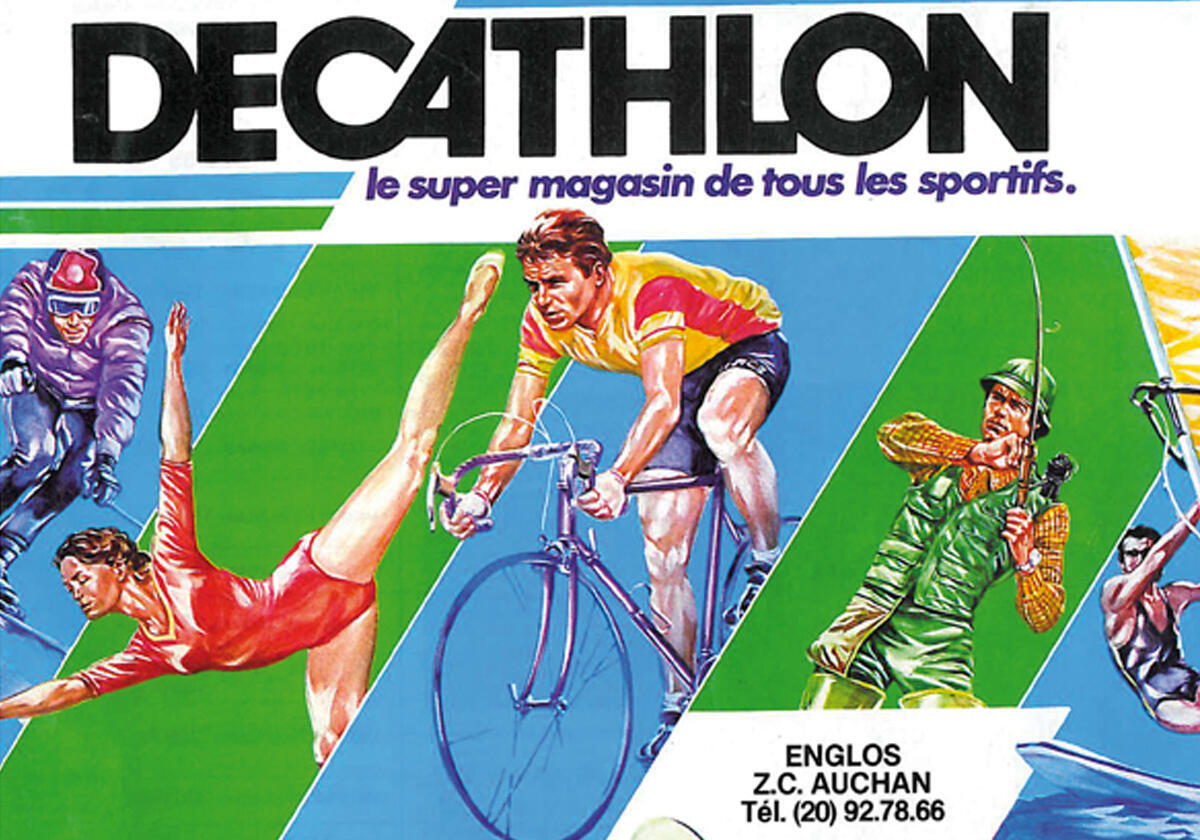The image is a highly detailed and colorful magazine cover centered around various sports activities. At the top, in bold black letters, it reads "Decathlon." Below that, in blue text, is the French phrase "Le Super Magasin de Tous les Sportifs," suggesting a comprehensive sports store. The cover is divided into five distinct panels, alternating between blue and green backgrounds.

On the far left, against a blue background, is an artistic rendering of a skier navigating down a mountain slope. Next to this, against a green background, is a female gymnast in a red leotard, striking a pose with her legs extended and arms outstretched. The central panel, also in blue, features a male cyclist wearing a yellow shirt with a red stripe, pedaling vigorously on his bicycle. In the fourth panel, against a green background, there's a fisherman dressed in a green vest and a yellow checkered shirt, holding a fishing rod as if battling a catch. Finally, the far-right panel, set against a blue background, displays a man in a blue shirt and shorts engaged in sailing.

Beneath the fisherman, the text "Inglos Zisi Aushan" is displayed along with a telephone number, adding an element of contact. The overall composition effectively captures the essence of diverse sports and the vibrancy associated with each activity.